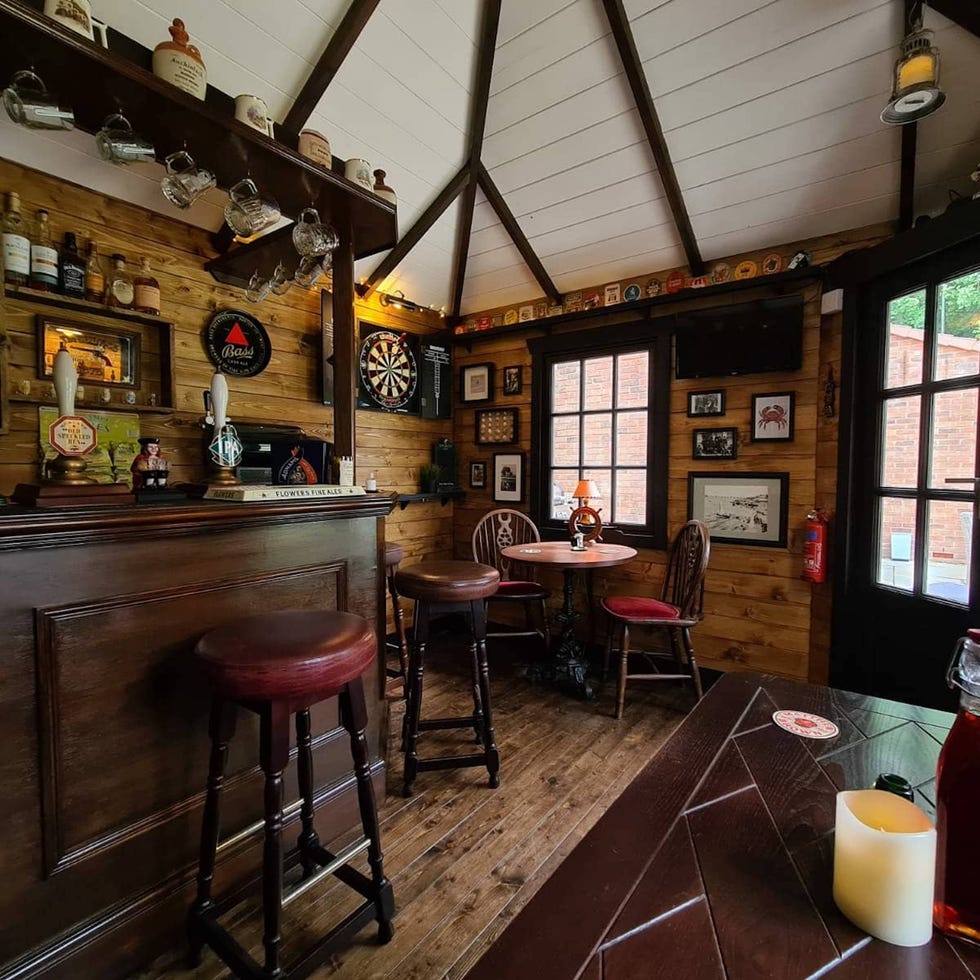The image depicts the inside of a cozy, intimate pub bathed in daylight. The rectangular room, slightly taller than it is wide, features a high ceiling with white planks and intersecting dark brown beams. The décor is predominantly rustic, with extensive wood paneling throughout the walls and floor, and a high, fully wooden bar located on the left side. The bar is adorned with a variety of jugs and beer steins, as well as numerous liquor bottles and hanging glasses.

To the right, there is a fancy wooden tabletop with intricate designs that holds a whitish candle. Nearby, a set of reddish-brown stools with black and red seats are arranged, and further in the back, a round table is surrounded by elegant brown chairs with red felt padding. Images and signs fill the walls, adding to the pub's charming décor. Additional tables are scattered throughout, with one in the back corner.

A dartboard featuring a red, black, and white design is visible in the back, along with a small flat-screen TV. The back door and a window allow natural light to filter in, giving a glimpse of the exterior brick buildings. The pub also has practical touches like coasters, drink coasters, and even a fire extinguisher near the front door. Overall, the bar exudes a warm, old-world charm, reminiscent of a neighborhood tavern.